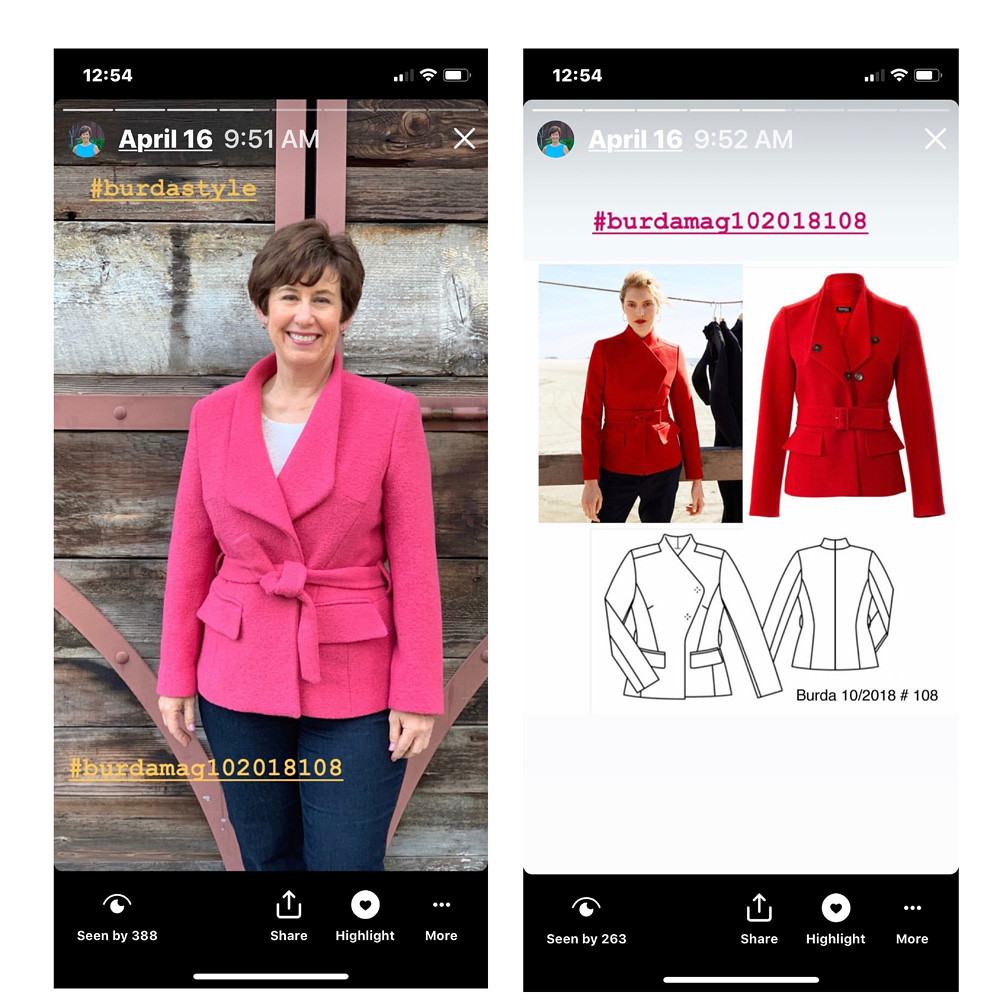The image consists of two Instagram Reels screenshots, captured on April 16th. The first screenshot, taken at 12:54 PM, features a middle-aged woman with short brown hair wearing a felt pink jacket and blue jeans, standing in front of a wooden background and possibly reflecting windows with trees. Yellow text at the top and bottom of the image displays hashtags: #birdaStyle and #birdamag102018108.

The second screenshot, taken a minute later at 12:55 PM, showcases a model with blonde hair in a bright red jacket and black pants. Just below the photograph, there is a black-and-white hand-drawn sketch of the jacket. The pink text hashtag #birdamag102018108 is visible again in this image, further linking both screenshots through the similar fashion theme.